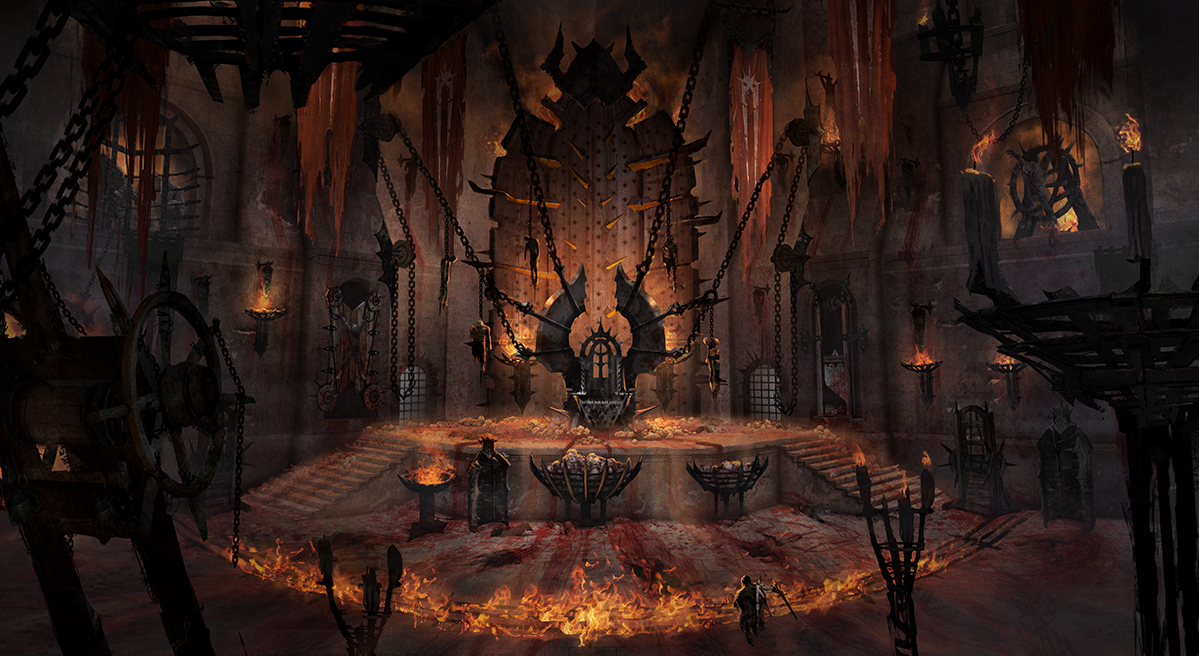In this computer-generated illustration, we find ourselves in a vast, dark, and eerie dungeon-like setting that seems reminiscent of a scene from a video game. The entire area is cast in deep, shadowy hues of black, brown, and gray, with the surroundings filled with jagged rocks and dimly lit by numerous torches burning fiercely on stands and walls. In the center of this foreboding space stands a large rock pillar, crowned by an imposing throne with two gigantic black wings extending vertically above it, giving an impression of immense power and menace. The throne rests on a stage encircled by a ring of blazing fire, enhancing the sinister atmosphere. 

Two sets of stairs ascend to the stage from either side, leading up to what could only be described as the centerpiece of the scene. Chains are omnipresent, hanging from the walls, linked to various pieces of old wooden machinery with large spokes and wheels, and connected to a complex system of pulleys. These chains and the metal implements embedded in the walls, looking like sharp thorns, contribute to the dungeon's grim aesthetic. Additionally, metal hooks and pits filled with rocks add further to the chaotic and menacing environment. This intricate and richly detailed scene conveys a powerful sense of danger and mystery.